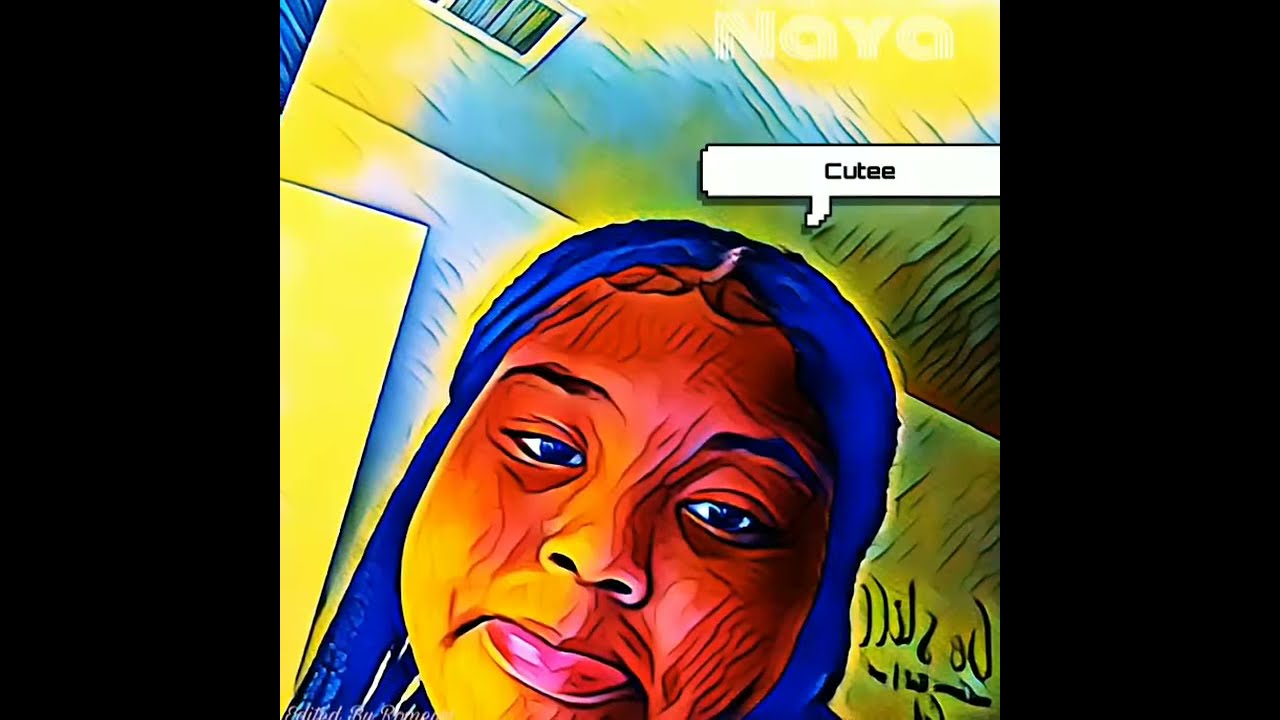This vibrant, pop-art style illustration presents a young African-American woman with a striking, digitally-edited appearance that mimics cartoon colorization. Her hair is a glowing dark blue with a yellow aura, framing her face which combines red, brown, and yellow tones. Her lips are a mix of pink and purple, and her eyes are brown beneath black eyebrows. The expression on her face is a slight frown. She is situated in a room with a ceiling that has a white vent and walls painted in shades of green, blue, and yellow. Above her head is a white conversation bubble containing the word "CUTE" spelled out as "C-U-T-E-E." The square-format image is inset into a black landscape background, featuring a white-screened logo "N-O-Y-O" in the top right corner and mirrored script on the bottom right, adding to the modern, graphic feel of the artwork.